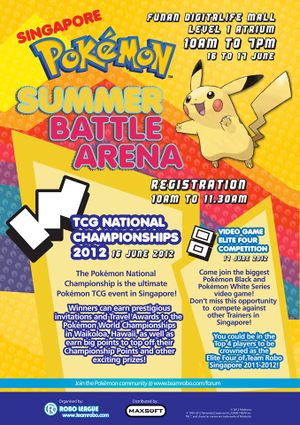The image features a vibrant and colorful background blending shades of yellow, orange, red, purple, blue, and dark blue. In the upper left corner, red text reads "Singapore." Directly below, the words "Pokemon Summer Battle Arena" are displayed in a striking combination of yellow and blue.

In the upper right corner, white block text announces the event location and details: "Funan Digital Life Mall. Level 1 Atrium. 10 a.m. to 1 p.m. 16 to 17 June."

Below this information, a cartoon character resembling Pikachu captures attention with its iconic yellow color and long, bunny-like ears. Further down in white block text, the caption reads: "Registration 10 a.m. to 11:30 a.m. TCG National Championships 2012. 16 June 2012." In blue text, an additional note emphasizes the significance of the event: "The Pokemon National Championship is the ultimate Pokemon TCG event in Singapore."